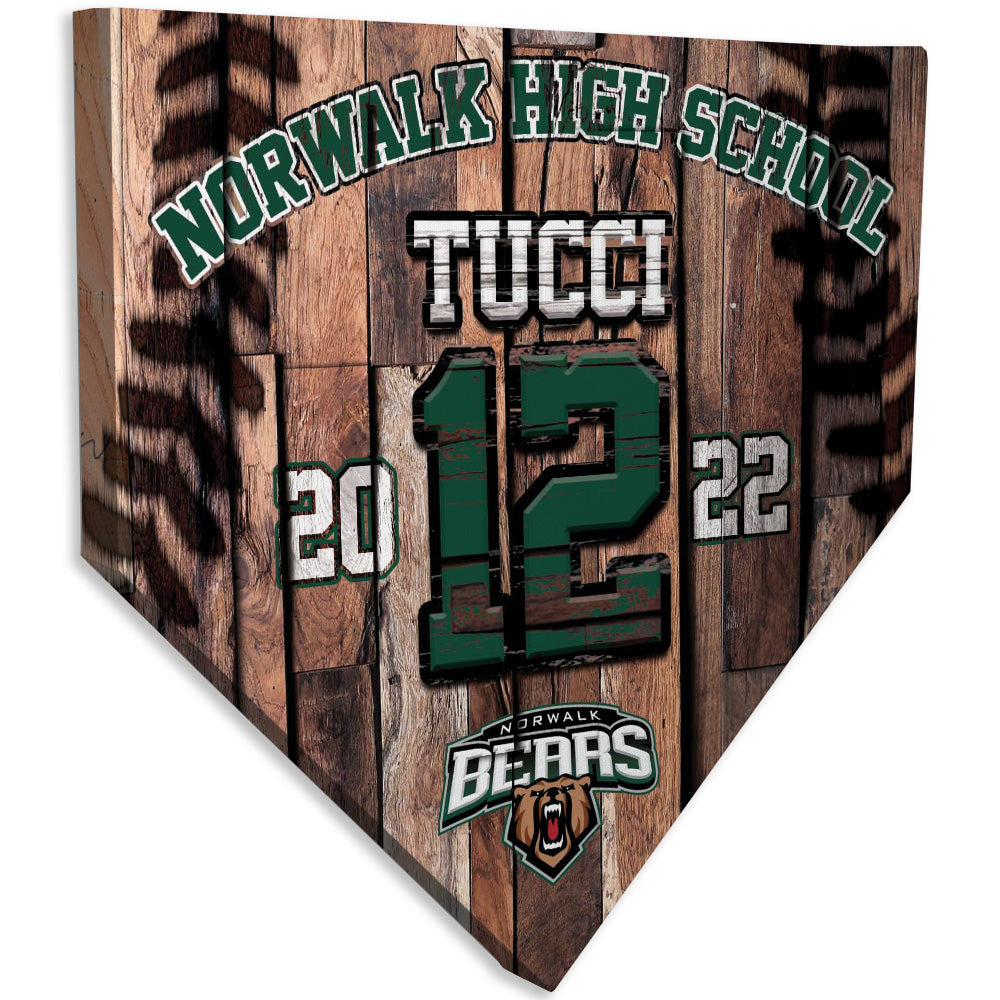The image features a rustic, wood-grain sign in the shape of a home plate, resembling a stylized award or commemorative plaque. At the top of the sign, "Norwalk High School" is prominently displayed in large green letters with a white and black border, evoking the classic varsity font. Directly below, in bold white letters, is the name "Tucci," flanked by the large green number 12, which also has a black outline. On either side of the number 12, the years "20" and "22" appear in white letters, outlined in black and green, forming the complete year "2022." Towards the bottom, "Norwalk Bears" is inscribed in green, black, and white text next to an illustrated roaring bear. The wooden sign, which has a distinctive blocky appearance reminiscent of a rustic butcher block, also features intricately burned baseball stitches on the left and right edges, adding to its unique, sporty aesthetic. The image captures the detailed craftsmanship and pride associated with Norwalk High School and its baseball team, the Norwalk Bears.